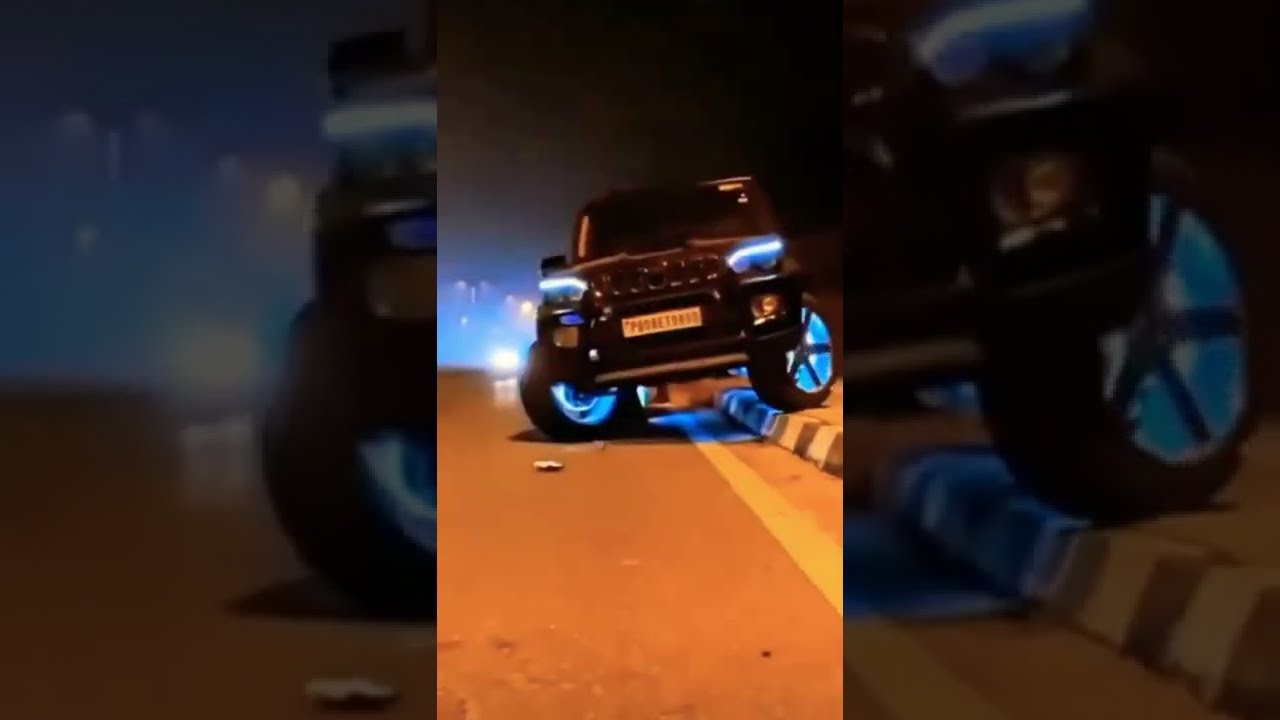The image features a large, black SUV, resembling either a Land Rover or Jeep, positioned predominantly at the center. The SUV's custom-made tires are equipped with striking neon blue lights that illuminate the surroundings, particularly evident where the vehicle is interacting with the curb. This scene is captured at night, evidenced by the darkened backdrop and the light sources. The vehicle appears to be transitioning from the curb back onto a gray road, which is marked by a white line. The license plate on the SUV suggests it is from a foreign country, indicated by its distinct yellow coloring and format. Tinted windows add to the vehicle's imposing appearance. The distant background includes minor traffic activity, hinting at an urban setting. The overall image emphasizes the SUV with its vibrant blue-lit tires and gives off an air of dynamic movement.